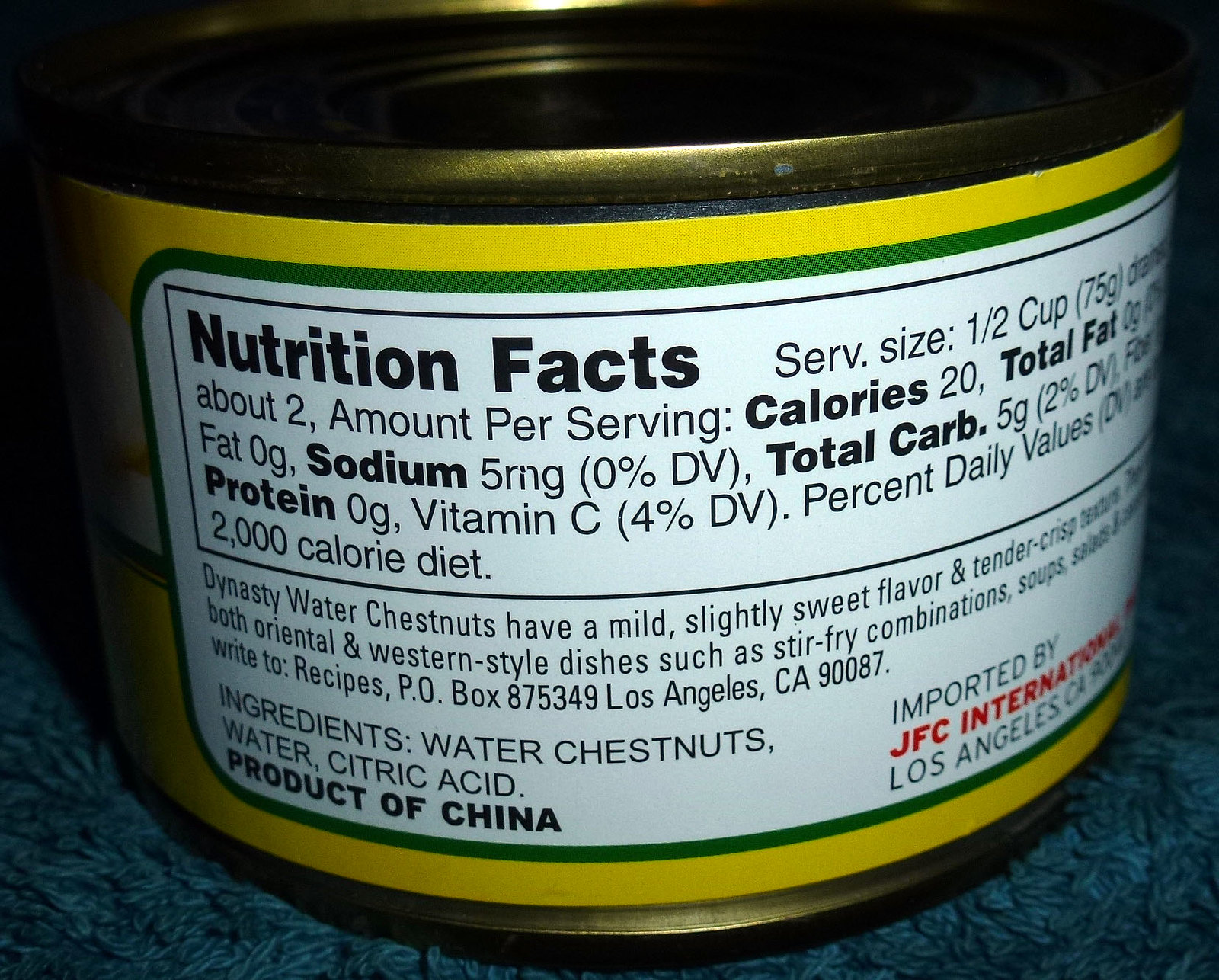The image showcases a close-up of a can with elegant gold trim adorning both the top and bottom edges. The focus is on the detailed nutritional label on the back of the can. The label is headed by "Nutrition Facts" and specifies a serving size of 1½ cups (7 grams). Each serving contains approximately 20 calories. The nutritional breakdown per serving is as follows: Total Fat - 0 grams, Sodium - 5 milligrams (0% Daily Value), Total Carbohydrates - 5 grams (2% Daily Value), Protein - 0 grams, and Vitamin C - 4% Daily Value. The label continues to enumerate all the included ingredients, providing comprehensive nutritional information for the consumer.